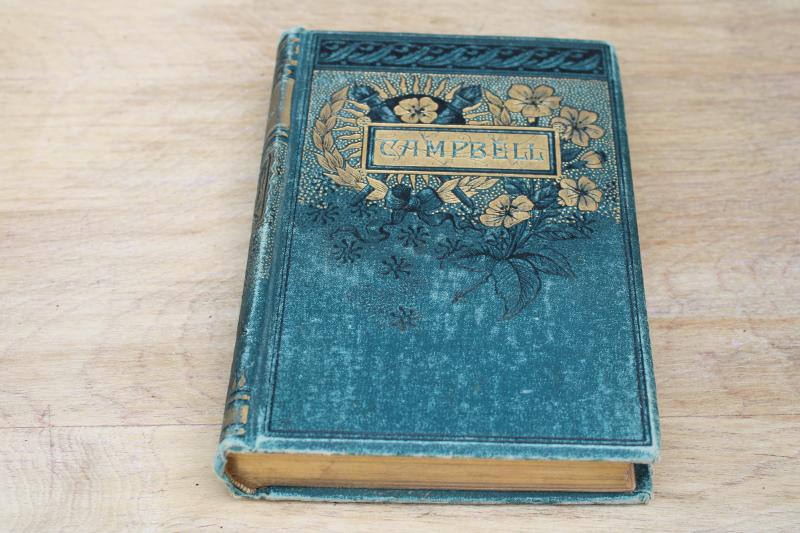The photograph captures a horizontally aligned rectangular image of an old hardback book resting on a scratched, light-colored wooden surface, which could be a floor, counter, or table. The book itself is faded blue, with its cover appearing worn and mottled, perhaps made of suede or fabric. A distinctive gold-embellished braid pattern crosses the top of the cover. Central to the cover is a shaded gold rectangle containing the word "CAMPBELL" in all capital letters. Surrounding the rectangle, golden floral designs and leaves adorn the right and left sides, along with a circle emitting gold rays, possibly symbolizing a sun. Below the middle of the cover, dark blue flower outlines add to the ornate design. The book's pages are noticeably browned and stained, indicating its age, though the spine is partially visible and appears aged as well.